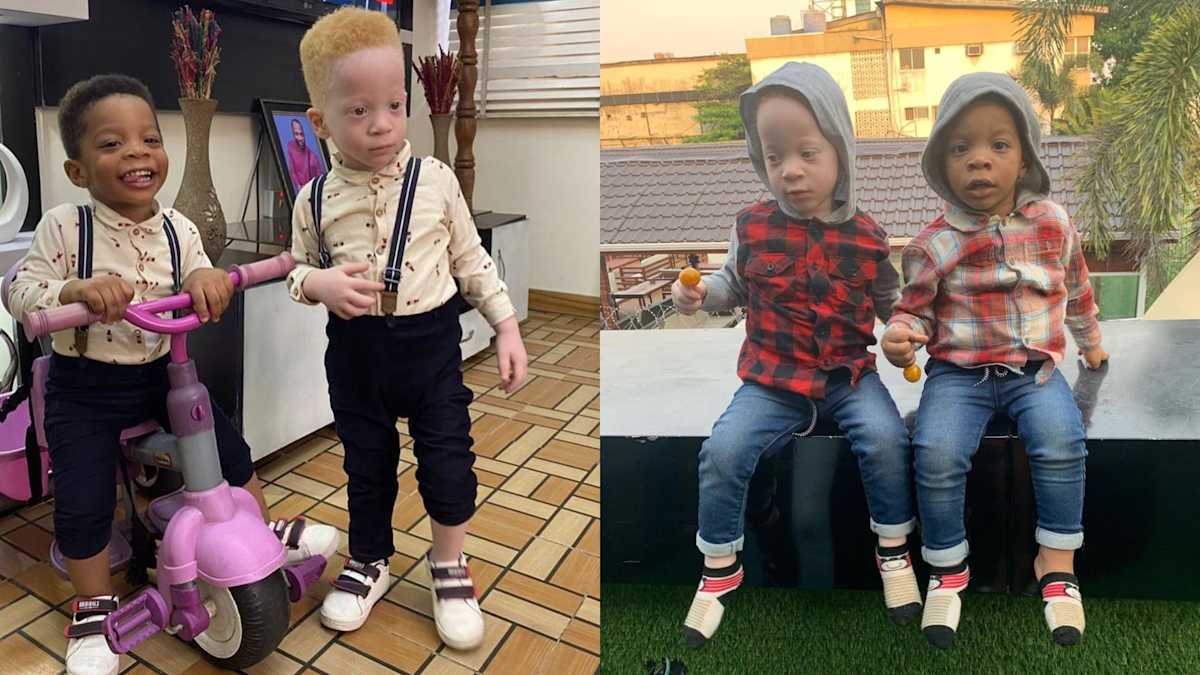This set of two detailed photographs features the same two young boys, one African American and the other Caucasian, possibly siblings with Down syndrome. In the left image, set indoors on a brown tiled floor with Venetian blinds in the background, the African American boy is riding a purple tricycle. He is dressed in dark pants, black suspenders, a cream-colored shirt with a dotted pattern, and white shoes with purple Velcro straps. Beside him, the Caucasian boy, who is very fair-skinned with red hair, stands in an identical outfit, both appearing playful. A table with vases, plants, and a framed photo can be seen behind them.

In the right image, the boys are outdoors, sitting on a bench against a backdrop of brightly colored houses with red, orange, and off-white hues and inclined gray roofs, with part of a tree visible. Both boys are now dressed in blue jeans, red, black, and white socks, and gray hoodies. The African American boy wears a plaid shirt, while the Caucasian boy, appearing fairer with a possible albinism trait, dons a buffalo plaid vest over his hoodie. Each child holds a small yellow sucker in one hand, with the African American boy also holding a small dinosaur toy, suggesting a moment of shared enjoyment and camaraderie.